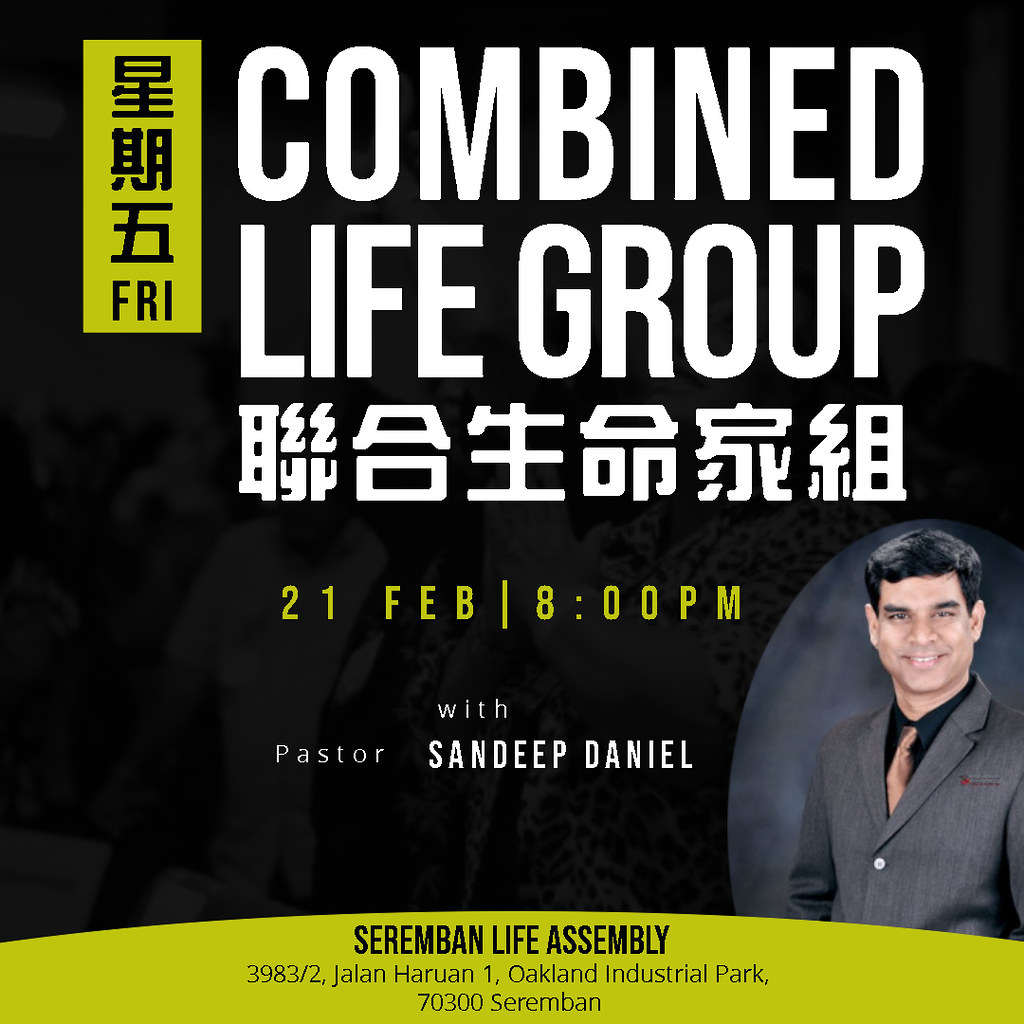This detailed infographic advertises a self-help seminar titled "Combined Life Group," prominently scheduled for Friday, 21st February at 8 p.m., featuring Pastor Sandeep Daniel. The background is primarily black and gray, with additional design elements including neon green and yellow accents. The header includes two lines of all-caps white block letters stating "Combined Life Group," followed by a row of white symbols that appear to be either Chinese or Japanese text. Below this, centered in neon green text, is the event's date and time, alongside the announcement of Pastor Sandeep Daniel's participation in white text. On the lower right, there is a photo of Pastor Sandeep Daniel, who appears to be in his late 30s to early 40s. He has short black hair, is smiling, and is dressed in a gray suit, black button-up shirt, and a bronze-colored tie. The bottom section of the image, shaded in neon green, provides the venue details, "Seremban Life Assembly," along with the address: 3983/2 Jalan Haruan 1, Oakland Industrial Park, 70300 Seremban. Additionally, a neon yellow rectangle on the left side of the image contains black symbols and the abbreviation "FRI," indicating the day of the week. The overall design provides a clear, engaging notice for the upcoming seminar.